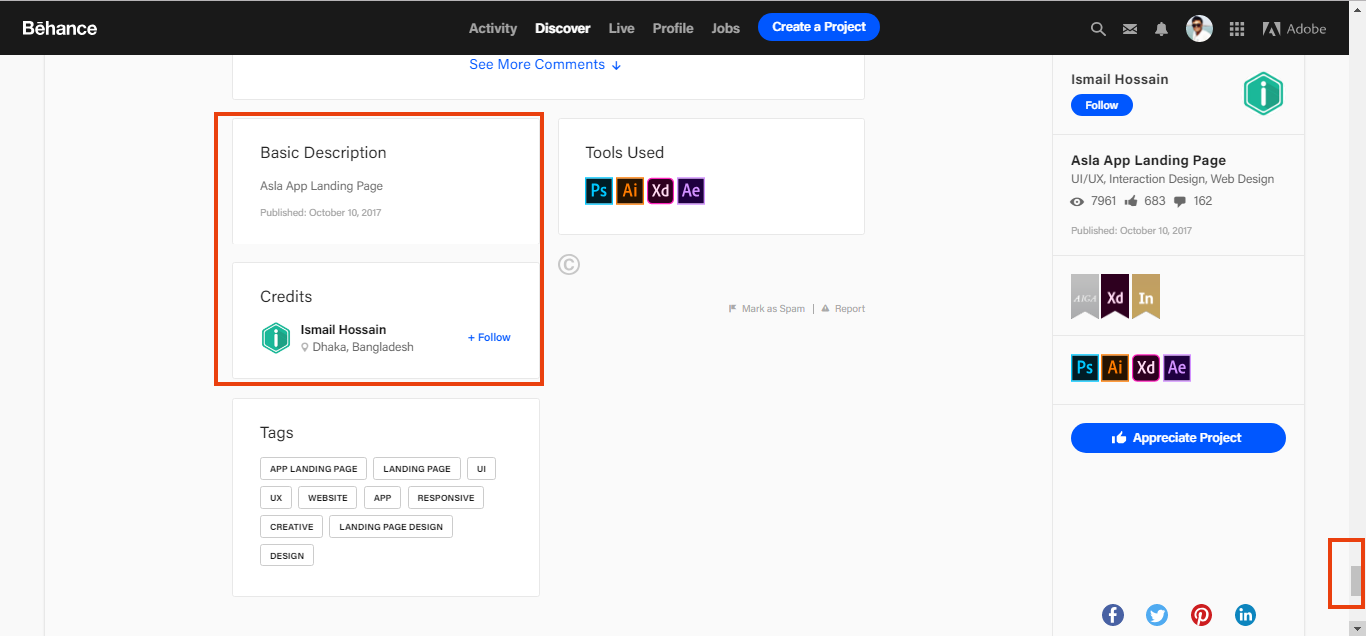This image depicts a detailed view of a Behance project page dedicated to the AJA app landing page, published on October 10th, 2017. The interface is organized with several sections: 

- At the top, there are navigation tabs labeled "Activity," "Discover," "Live," "Profile," "Jobs," and "Create a Project" highlighted in blue, indicating its affiliation with Adobe.
  
- Below is a basic description box, detailing the project name "AJA app landing page" by Ismail Hazem from Bangladesh, with a blue follow button for Ismail on the right.

- Under the description, a series of tags summarize key themes and components such as "app landing page," "UX/UI," "website," "app," and "responsive design."

- Adjacent to the description is a "Tools Used" section, represented by icons like Photoshop (PS), Illustrator (AI), Adobe XD (XD), and After Effects (AE), styled as periodic table elements.

- On the far right, alongside Ismail Hazem's name is another clickable follow button.

- The lower section expands into details about the app landing page, with categories like "interaction design" and "web design." Metrics for views, likes, and comments are visible, alongside an "Appreciation Project" button for further exploration, shaded in blue.

The overall layout provides a comprehensive view of the project’s essentials, including author credits, description, tools used, and engagement statistics.